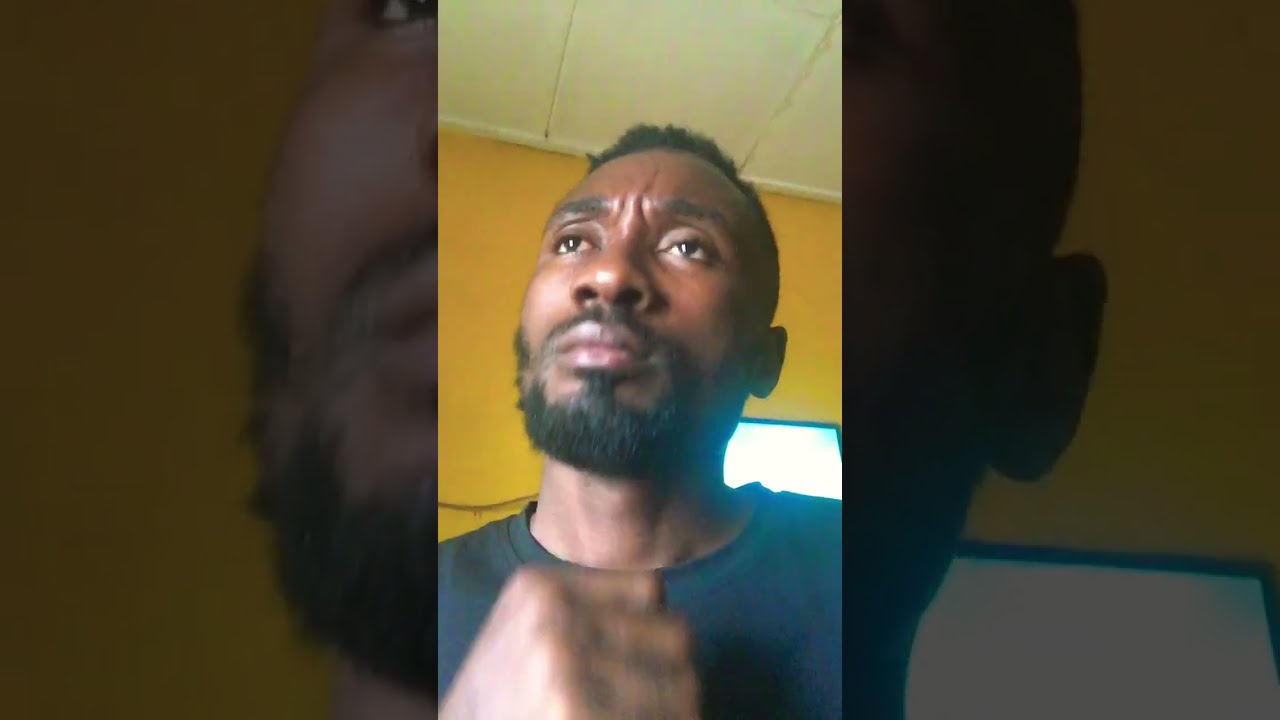This image features an up-close, slightly blurry shot of an African-American man set against a background with a distinctive layout. The central image is brightly lit and displays the man from the top of his head to his chest, with his clenched hand held close to his chest. He looks serious, possibly upset or contemplative. The man's features include a short hairstyle, a goatee, and a mustache. He is wearing a blue shirt, which might be a sweatshirt.

Surrounding this central image are zoomed-in segments of the same picture on both the left and right sides, presented in darker tones. The background includes a white ceiling and yellow wall. A glowing television or screen is visible over the man's shoulder, casting some light. The zoomed-in portions on the sides capture details like parts of his face, ear, lips, and portions of the room's elements, enhancing the depth of the overall image. There is no text present anywhere in the picture, and there are no other people visible. The man appears to be looking slightly upwards and towards the top left.